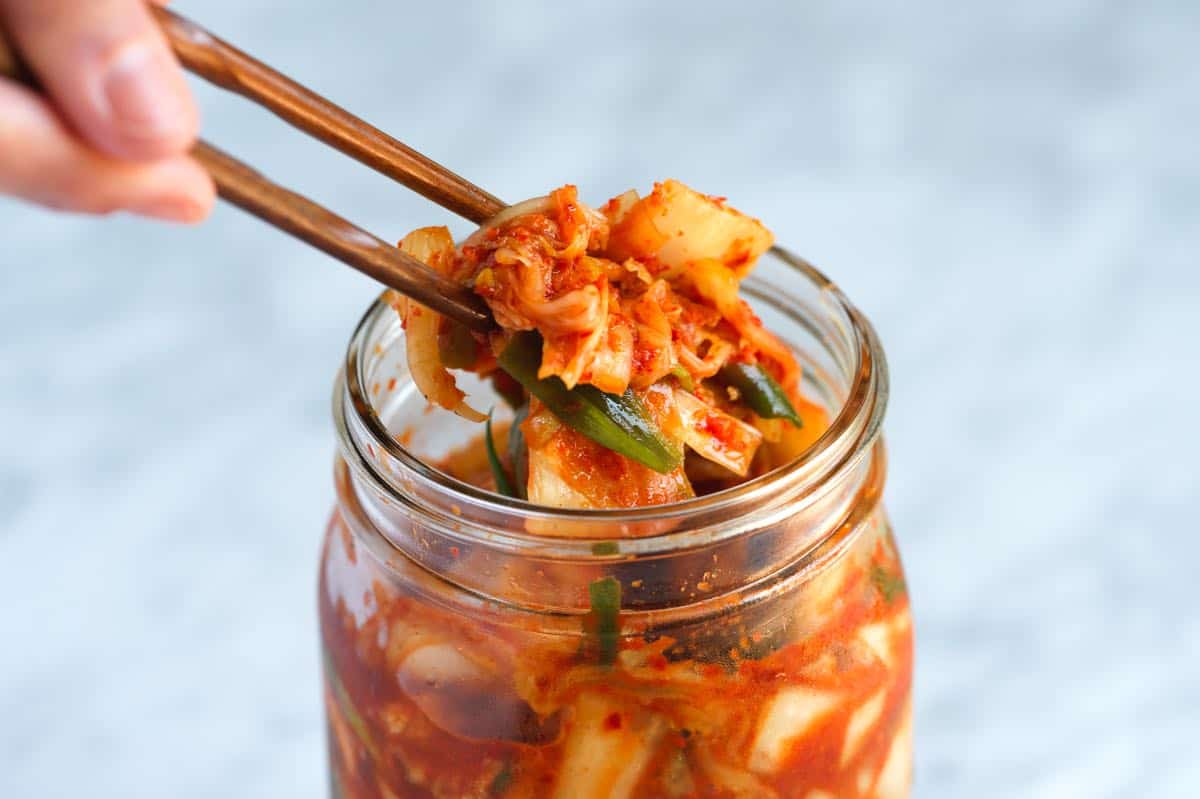In the photograph, a clear glass jar, potentially a mason jar with a slightly square body and a round, screw-on cap (not visible), contains a mix of food items. The contents appear to be kimchi, with typical kimchi ingredients such as cabbage pieces (both whitish and greenish), immersed in a red brine with visible red spice flakes. A hand in the upper left corner of the image, which could belong to a person of any descent, is using two brown wooden chopsticks to lift a piece of this mixture from the jar. The background is blurred and features light, indistinct shades of white, gray, and a very light blue, possibly indicating a countertop or wall.